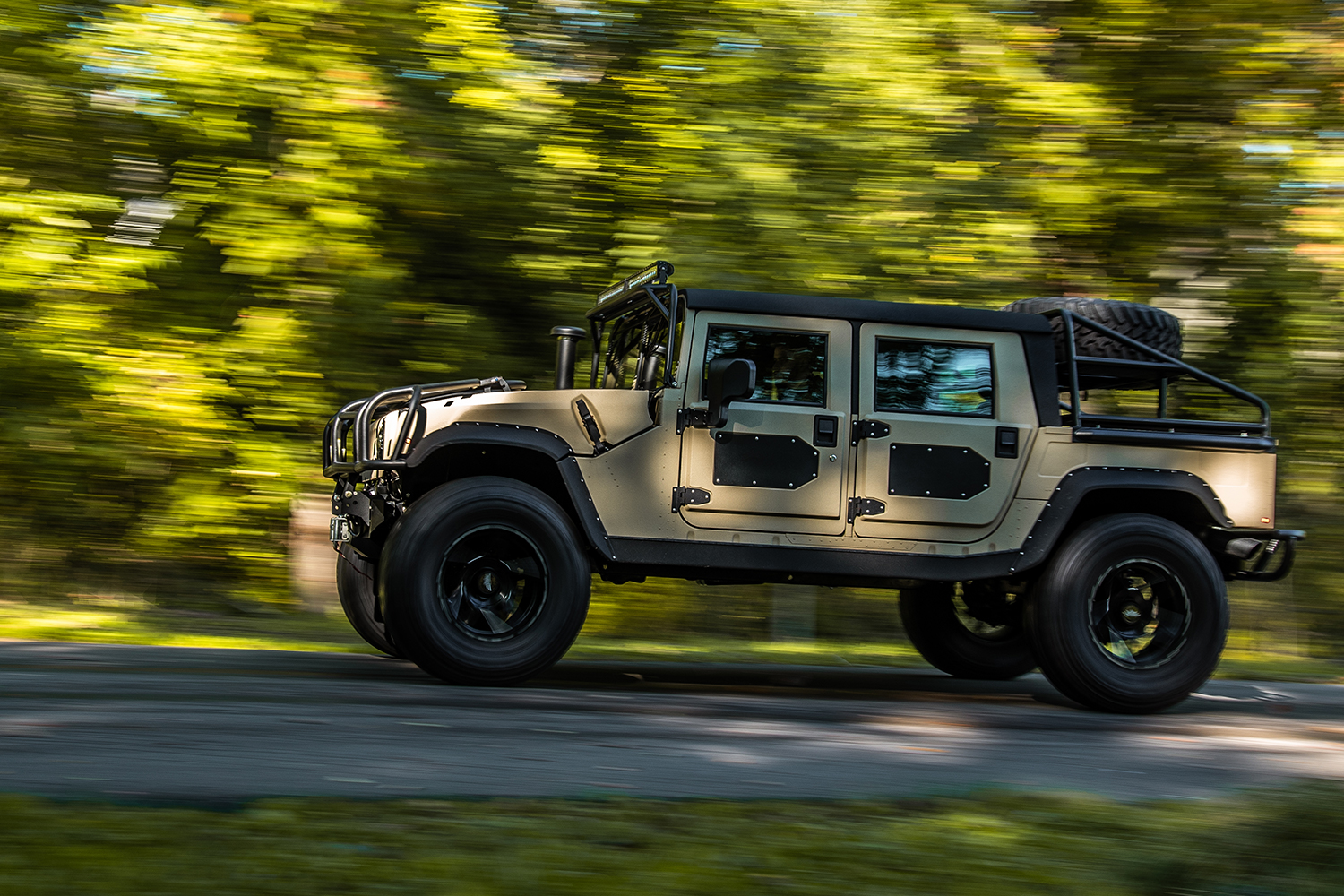This image captures a tan or creamy bronze jeep-like vehicle, possibly a Humvee or military-style jeep, driving rapidly on a road. The vehicle is sharply in focus, whereas the background, consisting of trees, road, and grass, is motion-blurred, indicating the vehicle's swift movement from right to left across the frame. The jeep features two front doors and a truck bed-style rear end, with a large, black spare tire mounted on a metal rack in the back. The vehicle's black trim accentuates its military aesthetic, and it is equipped with a metal bar and lights above the windshield, further enhancing its rugged, industrial look. This modern jeep, portraying an expensive, army-grade design, prominently displays black tires and rims, reinforcing its robust build.